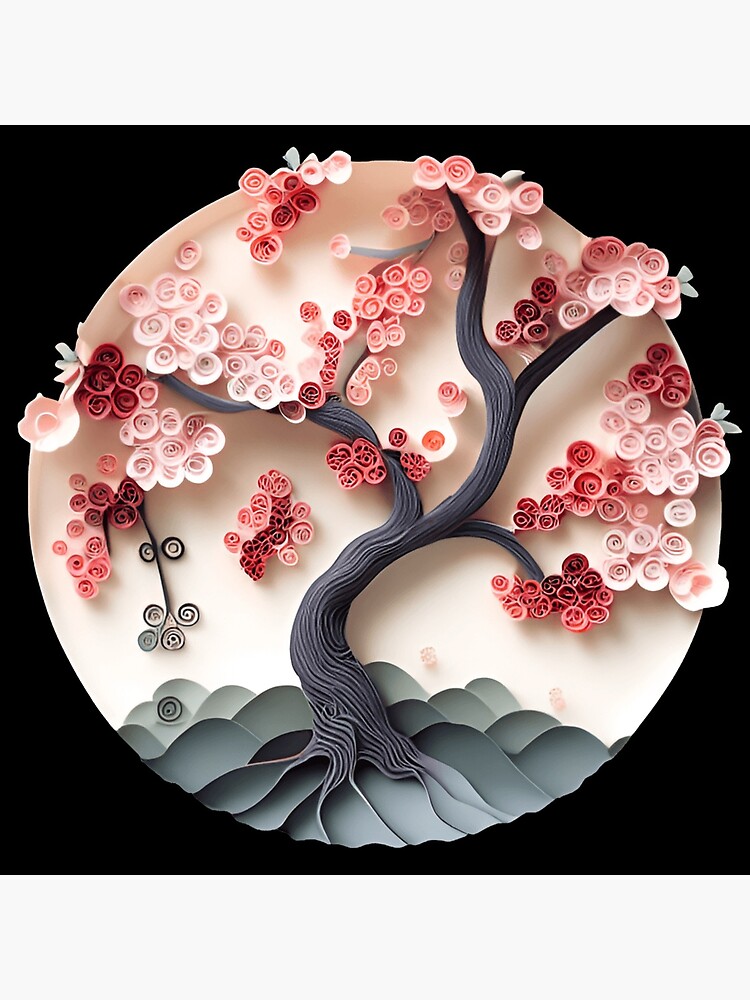In this artist's rendering on a circular, white background, we see an intricately detailed gray tree branch sprawling out and twisting like a bonsai tree, emerging from green wavy mounds near the bottom. The circle itself is set against a black backdrop, framed by a light pink border. The tree, evocative of a cherry blossom, diverges into multiple branches, each adorned with pink and white petals in varying shades. Some branches display clusters of these blossoms, while others appear to have pink flowers floating nearby, suspended in midair. Additionally, a few grayish sprouts extend beyond the circle’s edge on the right-hand side. To the left of the tree, a pink petal is captured in mid-fall, and at the upper left corner, more detached flowers and petals add to the dynamic composition of this piece.